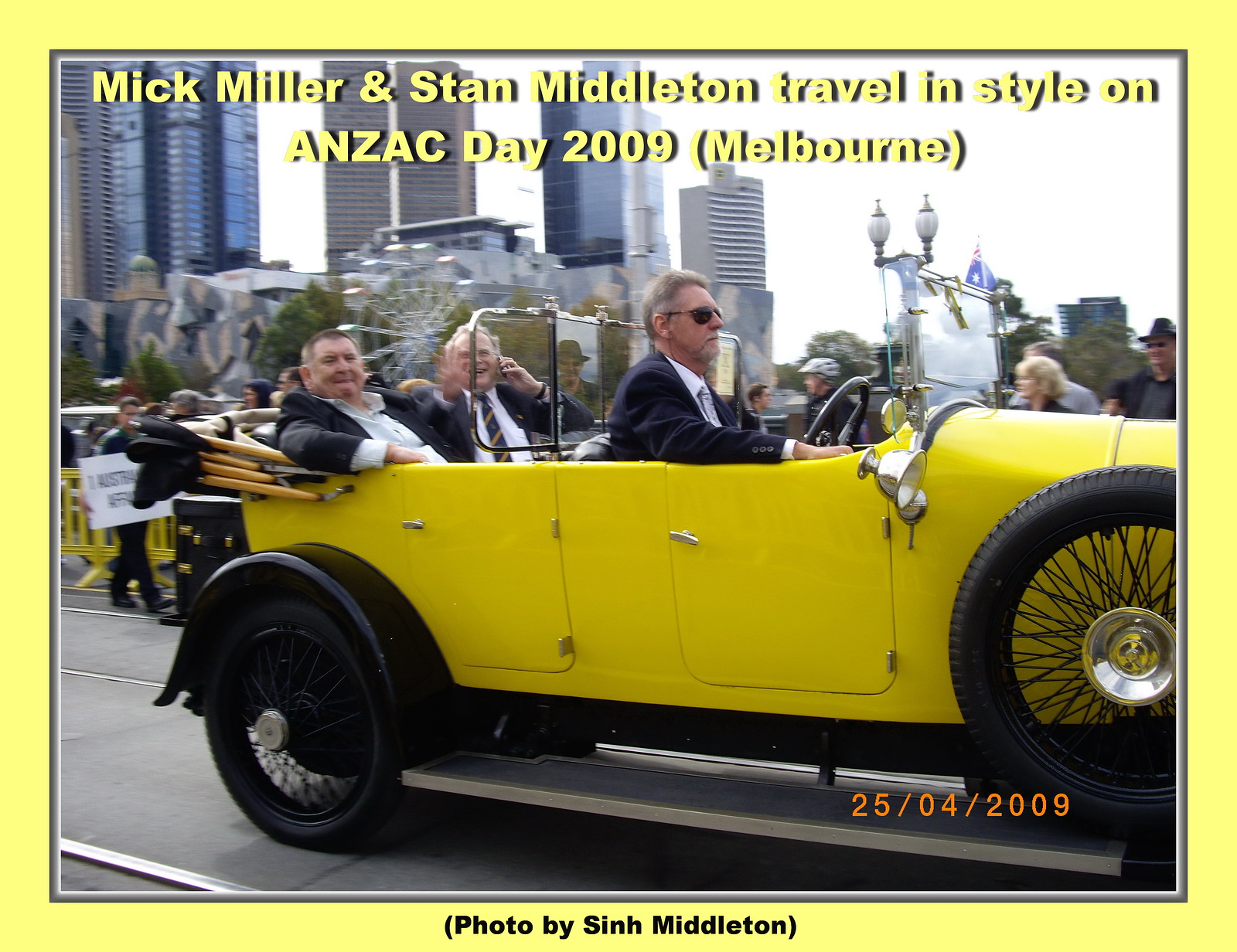Set against a vivid yellow backdrop, the photograph is intricately framed by a yellow border, creating a bold and striking visual. Within the image, three Caucasian men are seated in an antique yellow car whose top is down, symbolizing a ride through a memorable cityscape. The vehicle is driven by a professional-looking man donning sunglasses, seated on the right side, indicative of European car designs. Behind him, two men in blazers and button-down shirts sit in the back seat, one of whom appears to be on the phone and waving at the camera. The trio is likely Mick Miller and Stan Middleton, as referenced by the yellow text at the top of the photo that reads, "Mick Miller and Stan Middleton travel in style on ANZAC Day 2009, Melbourne." This text, along with the date "25/04/2009" inscribed in orange in the bottom right corner of the photograph, emphasizes the significance of the event and location. In the blurred background, a cityscape emerges, complete with towering skyscrapers, a Ferris wheel, and a crowd of onlookers behind a yellow fence, possibly marking a public gathering or celebration. The photo is credited to Sin Middleton, marked in black letters and parentheses beneath the picture.